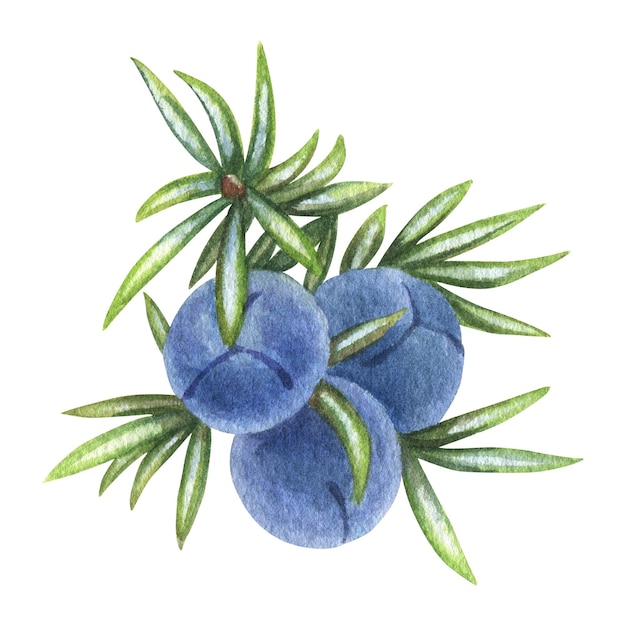The image depicts a simple, yet detailed, watercolor painting of three plump, in-season blueberries arranged in an upside-down pyramidal shape. Each blueberry features a distinctive crease in the form of an upside-down Y. Surrounding the blueberries are multiple green leaves with pine needle-like textures, and some of these leaves have white centers and brown tips, hinting at where new growth might emerge. The painting is isolated against a stark white background, emphasizing the blue and green hues, and the art style is characterized by scratchy, faded textures that give a light, almost fuzzy appearance to the piece.